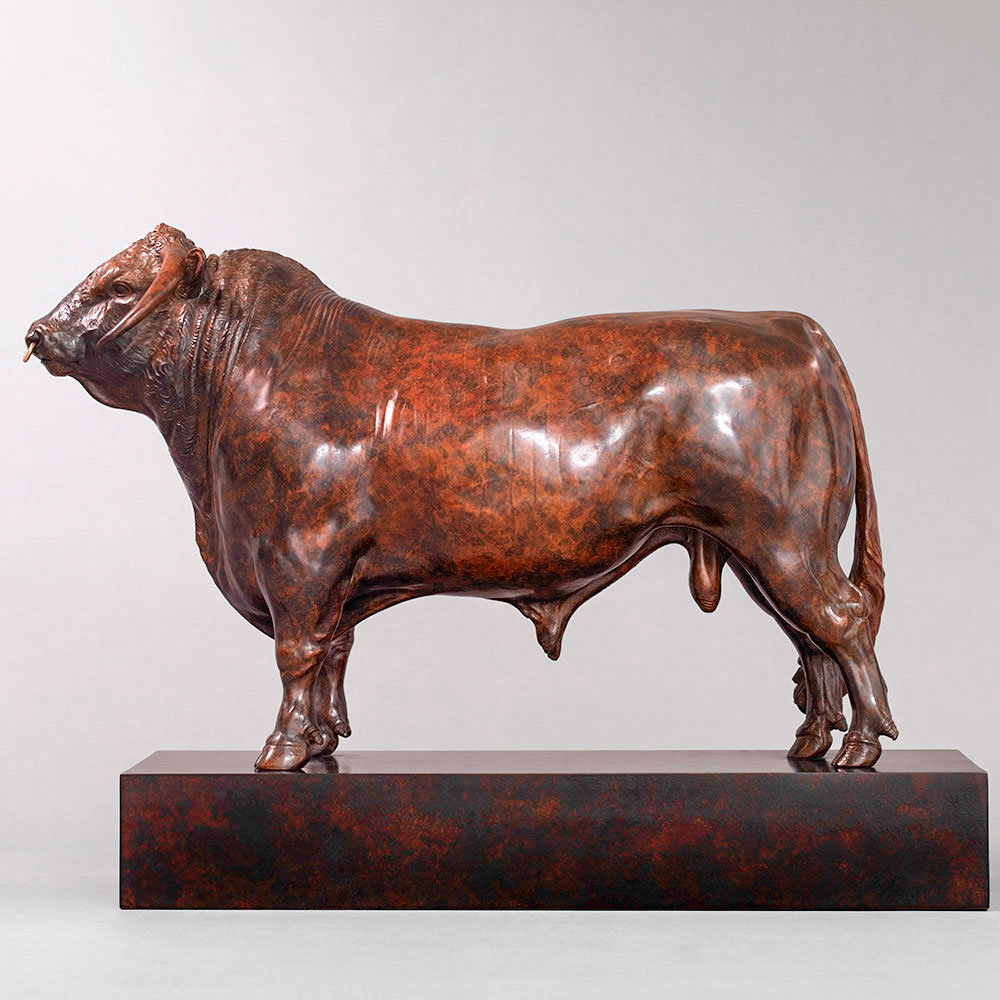This image features a detailed side profile of a bronze bull statue, standing on a sturdy, thick bronze base. The bull is facing left, its muscular frame accentuated by meticulous craftsmanship depicting ruffled skin and a prominent hunch behind its head. Its head, held high, displays a nose ring and downward-pointing horns on either side. The statue's rich, brown, marble-like finish, resembling burl wood, varies in shades, adding to its realistic appearance. The bull's thick tail and four hooves are distinctly visible, enhancing its anatomical accuracy. The backdrop is a neutral gray, further highlighting the intricate details of this impressive sculpture.